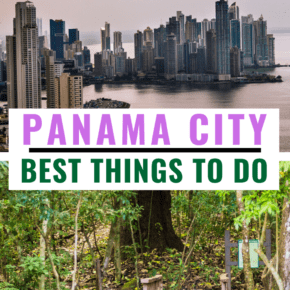The image is divided into two distinct sections. The upper portion showcases a breathtaking urban cityscape, captured during daylight hours. The skyline features a variety of buildings in shades of gray and tan, stretching from the lower left corner and curving around a body of water, extending nearly to the upper right corner. The sky above the cityscape displays a unique blend of grayish-pink hues, adding a dramatic effect to the scene.

The lower section of the image presents a natural contrast with the urban environment above. It focuses on the base of a large tree trunk, surrounded by a dense cluster of dark green saplings and low-lying plants, creating a serene, verdant setting.

Centrally positioned, against a white background, is a bold inscription in large, purple capital letters reading "PANAMA CITY," underscored by a solid black line that stretches horizontally across the image. Below this, in dark green text, are the words "BEST THINGS TO DO," providing a guide or recommendation within the context of the depicted locations.